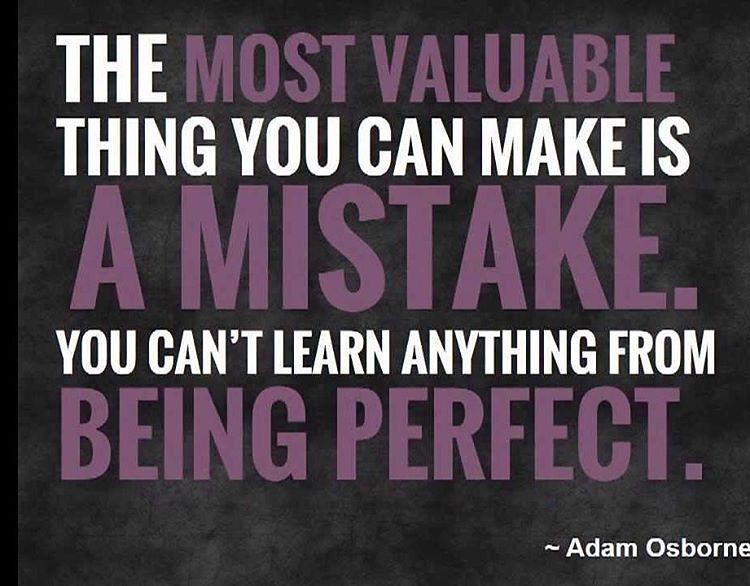The image features a close-up of an inspirational quote by Adam Osborne, set against a blackish-gray, splotchy background. The quote reads, "The most valuable thing you can make is a mistake. You can't learn anything from being perfect." The text is presented in a very large, bold font, with specific emphasis on certain words displayed in deep purple: "most valuable," "a mistake," and "being perfect." The remaining parts of the quote are in white and in a smaller font size. At the bottom right corner, the author’s name, Adam Osborne, is written in smaller white lettering. The entire quote is encased within a black border, enhancing the focus on the motivational message.